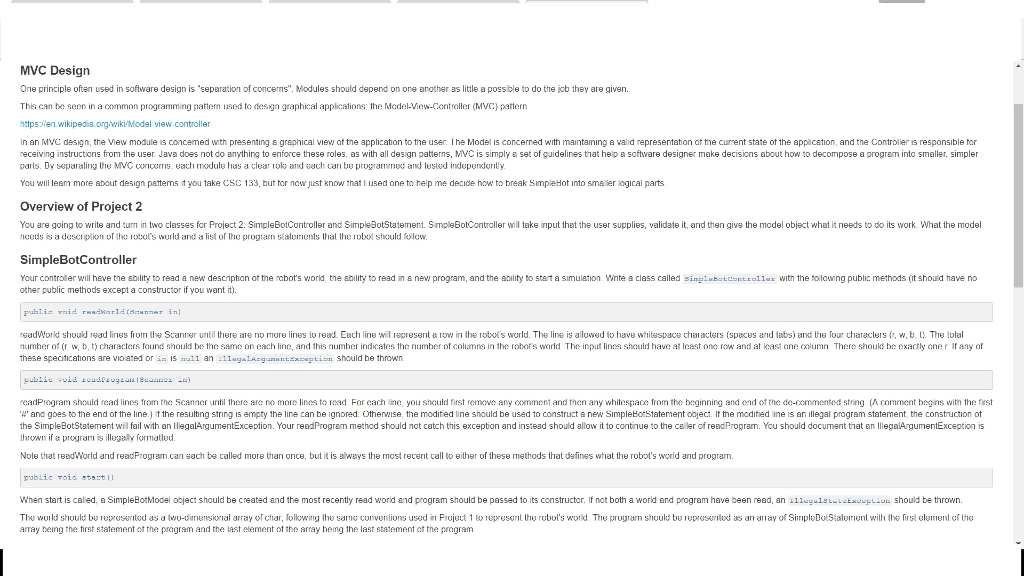A detailed screenshot from a computer screen predominantly showcases a plain white background with dark gray text, discussing the Model-View-Controller (MVC) design pattern in software and web development. The text starts by highlighting the principle of 'separation of concerns,' which emphasizes the importance of minimizing dependencies between different modules to achieve their respective functions. The content elaborates on the MVC pattern, focusing on how the 'View' component is tasked with presenting a graphical interface to the user. A notable detail is a succinct project overview, outlining the requirements for two classes, possibly for an assignment or project inception.

Additionally, the text features a description of a simple bot controller, detailing its capabilities to read new descriptions of the robot’s world, read new programs, and initiate a simulation. The screenshot also mentions public methods that can be utilized within this simple bot model. For further reading, a hyperlink to a Wikipedia page on the topic is included. Overall, this screenshot appears to be an instructional guide or project brief aimed at students or developers beginning their work on a software project utilizing the MVC design pattern.